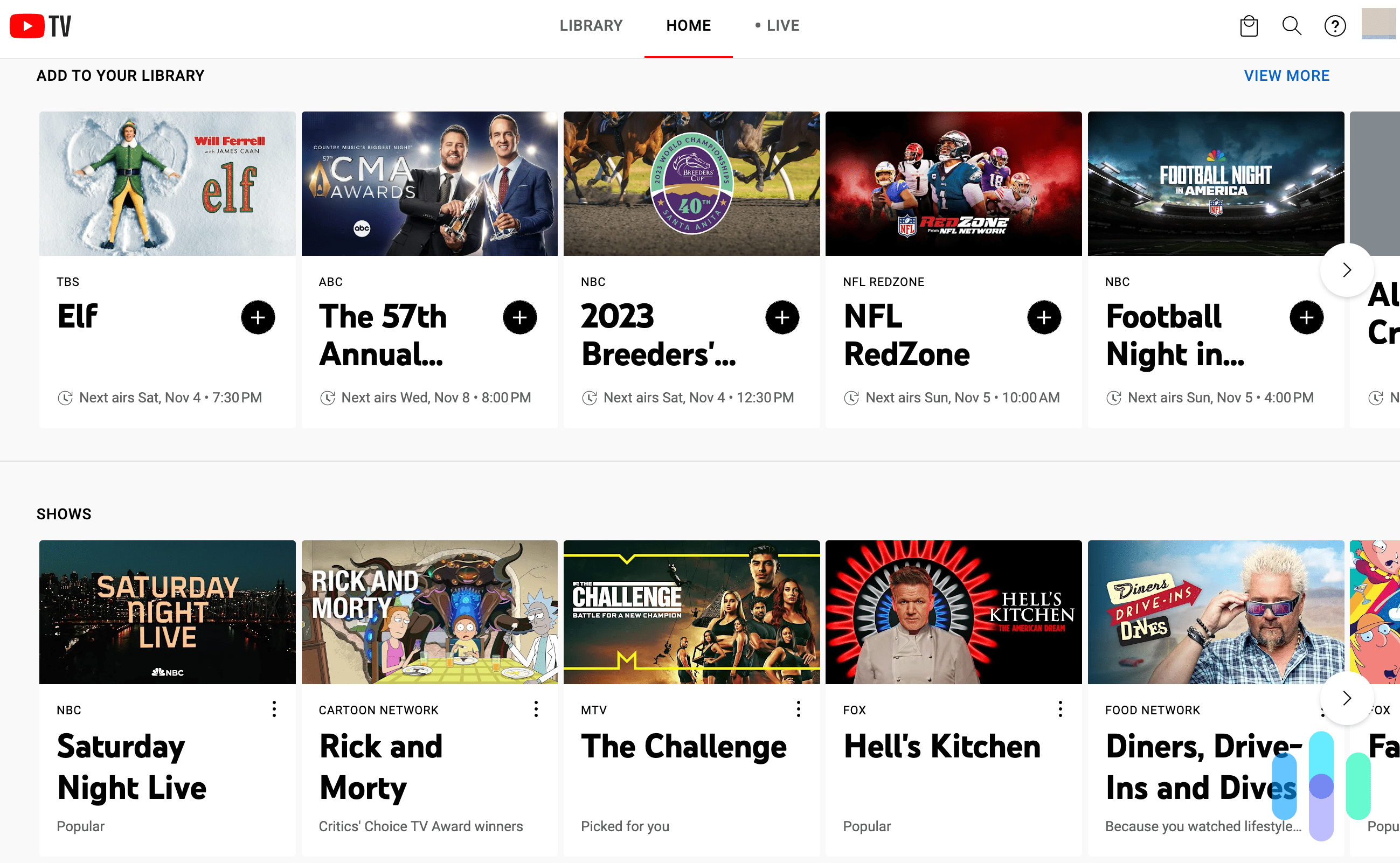The image is a screenshot of the YouTube TV webpage, showcasing various options to add to the user's library. In the top-left corner, the YouTube TV logo is prominently displayed. At the top center of the page, navigational tabs labeled "Library," "Home," and "Live" are clearly visible. Beneath the header, a call-to-action message reads "Add to Your Library," inviting users to enhance their viewing collections.

The content is organized into two main rows. The first row features movies and special events, starting from left to right: the movie "Elf," accompanied by a still from its poster; the "57th Annual CMA Awards"; the "2023 Breeders' Cup"; "NFL Red Zone"; and "Football Night in America." Each selection is visually represented by corresponding images or posters.

The second row highlights TV shows under the heading "Shows." From left to right, the selections include "Saturday Night Live," "Rick and Morty," "The Challenge," "Hell's Kitchen," and "Diners, Drive-Ins, and Dives." Each TV show is depicted with an image that represents the program, making it easy for users to identify and select their favorite shows to add to their library.